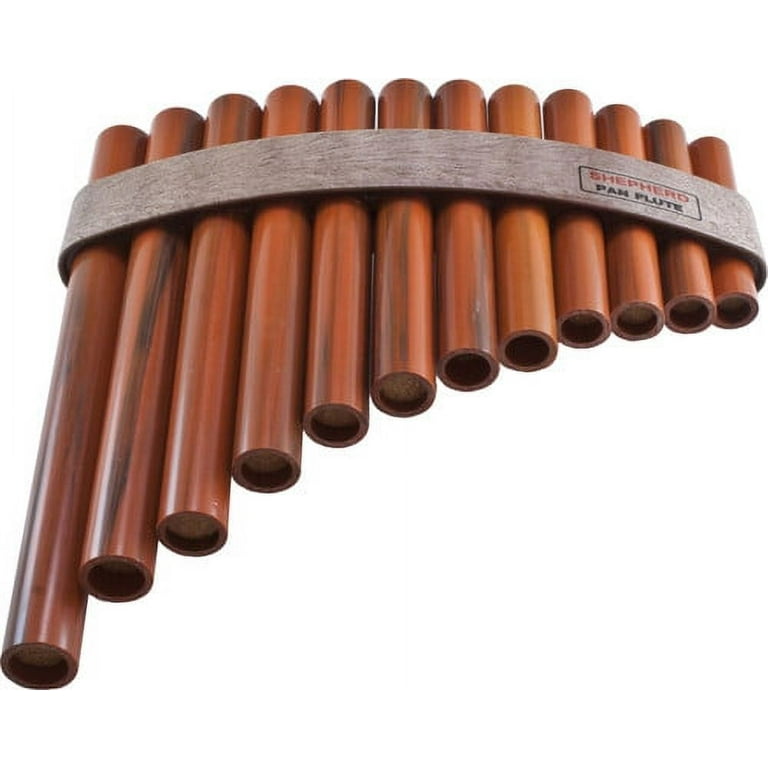This is a detailed close-up photograph of a pan flute featuring 12 cylindrical, hollow pipes of progressively decreasing lengths from left to right. The pipes are a glossy, mahogany, cherry-colored wood, with the grain visible, giving each pipe a slightly unique dark spotting. These pipes are fastened together with a light grayish-brown wooden band that wraps around them. This band, located towards the top half of the instrument, features text: “SHEPHERD” in red and “Pan Flute” in black, both encapsulated within a thin black rectangle with rounded corners. The instrument appears to have a lightly curved form, and the photograph is taken against a completely white background, suggesting it might be intended for an advertisement. The overall craftsmanship gives the impression of a finely polished, well-crafted musical instrument with a shiny, reflective surface.